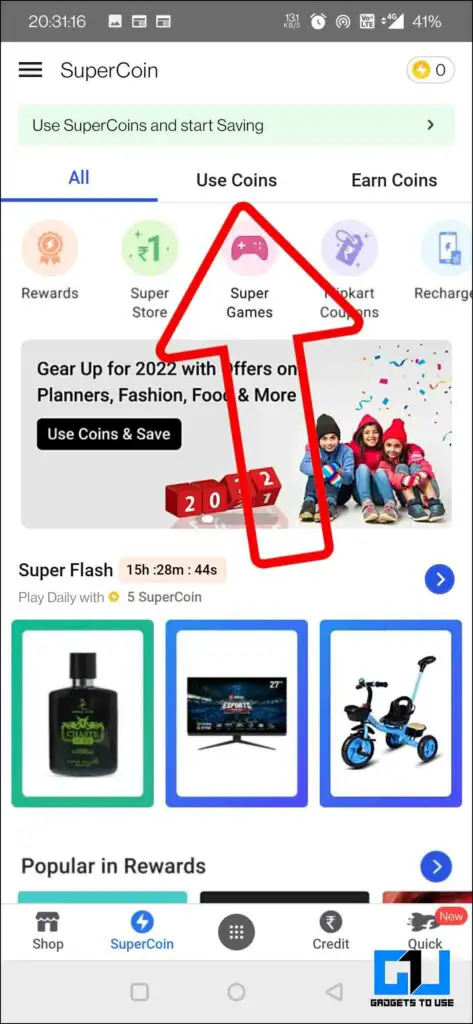The screenshot depicts a website interface on a tablet device. At the very top of the screen is a black status bar containing device information: the system time displayed as 20:31:13, various notification icons, a clock icon, a speedometer-like icon, a settings icon, full 4G signal strength, and a battery indicator showing 41%.

Immediately below, there is a blue banner featuring the SuperCoin logo along with the message "Use SuperCoins and start serving." Three tabs are visible: "All," "Use Coins," and "Earn Coins," with the "All" tab highlighted, indicated by a blue underline.

Below the tab section, there are several icons with accompanying text representing different sections:
- "Rewards"
- "SuperStore" (highlighted with a green button and the number 1)
- "SuperGames" (pinkish-red button displaying a game controller icon)
- "Flipkart Coupons" (marked by a price tag icon)
- "Recharge" (presumably for adding money or coins)

An arrow next to the "SuperGames" icon points toward the "Use Coins" section.

Following this, there's a promotional message: "Gear up for 2022 with offers on planners, fashion, food, and more. Use coins and save." Accompanying this message are three red dice displaying the numbers "2022" and an image of three children in winter attire—jackets, hats, sneakers, and jeans—seated on the floor.

Further down, the "SuperFlash" section shows a countdown timer with 15 hours, 28 minutes, and 44 seconds remaining, encouraging users to "Play daily with five SuperCoins." Below this are three product icons:
- A black bottle with green letters
- A widescreen TV labeled "27 inches"
- A blue tricycle with black seats and handles, featuring a grab handle for adults

The bottom section of the screen features the categories "Popular" and "Rewards," followed by navigation icons:
- "Shop" on the bottom left
- "SuperCoin" in blue
- A grid of nine dots in the center
- "Credit" and "Quick," with a red "Now" label next to "Quick."

Lastly, at the very bottom, the "Gadgets to Use" logo is displayed, confirming the brand name.